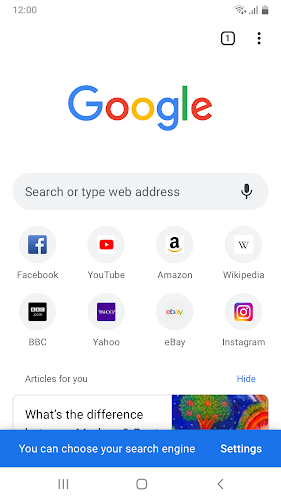The image displays a screenshot of a Google search screen on a cell phone. At the top left of the screen, the number "12" is visible, indicating the time. The top right corner features several icons: a Wi-Fi indicator, a service signal bar, and a battery indicator. Just below the status bar, there is a row showing the number of opened tabs (1) and a hamburger options menu.

Prominently positioned in the center is the Google logo in its signature multicolors. Directly underneath the logo, the text "Search or type web address" appears alongside a microphone icon for voice input. This section is displayed in dark text on a light gray background. Below this, there are two rows of icons and links encapsulated in circular "bubbles." The first row includes Facebook, YouTube, Amazon, and Wikipedia icons. The second row features BBC, Yahoo, eBay, and Instagram icons.

Further down, the screen displays "Articles for you" in gray text on the left, with a "Hide" option on the right. Partially visible is the title "What's the difference...", accompanied by an illustration of an apple tree. The text "You can choose your search engine" stands out in a white font on a blue background, followed by a settings icon. 

At the very bottom of the screen are navigational buttons. All these elements are situated on a light gray pop-out menu, set against a white background.